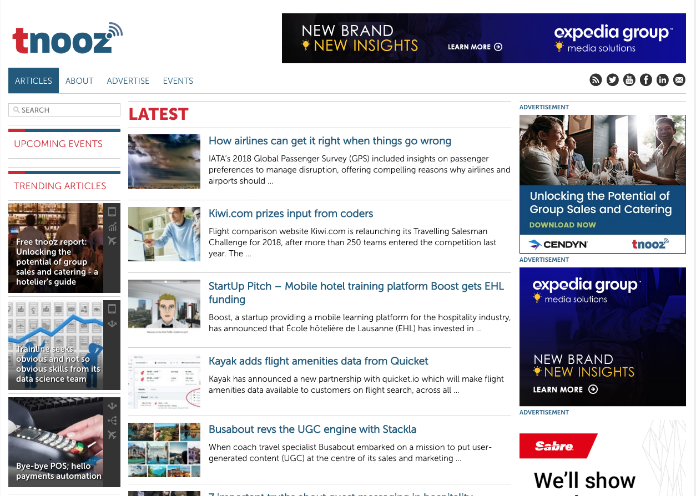This image captures a screenshot of the Tnooz website. The website's name "Tnooz" is displayed in all lowercase letters, with the 't' appearing in red and the 'nooz' in a teal color, alongside a radar-like graphic emanating from the text. The navigation menu at the top includes links for "articles," "about," "advertise," and "events," with "articles" currently selected.

The main content area is divided into several sections. The left side showcases the latest articles, highlighted by a red "latest" label. Each entry features a relevant image, a title, and a brief summary. For instance, one article depicts severe weather and is titled "How airlines can get it right when things go wrong," followed by a gray separator line and another article titled "Kiwi.com prizes input from coders."

On the right side, there are various advertisements. These include promotions for unlocking the potential of group sales and catering, an Expedia Group ad, and another partially visible ad from Sabre that states "we'll show" before being cut off.

Overall, the layout effectively organizes trending topics, stock market updates, and upcoming events, ensuring users can easily access a broad range of information.